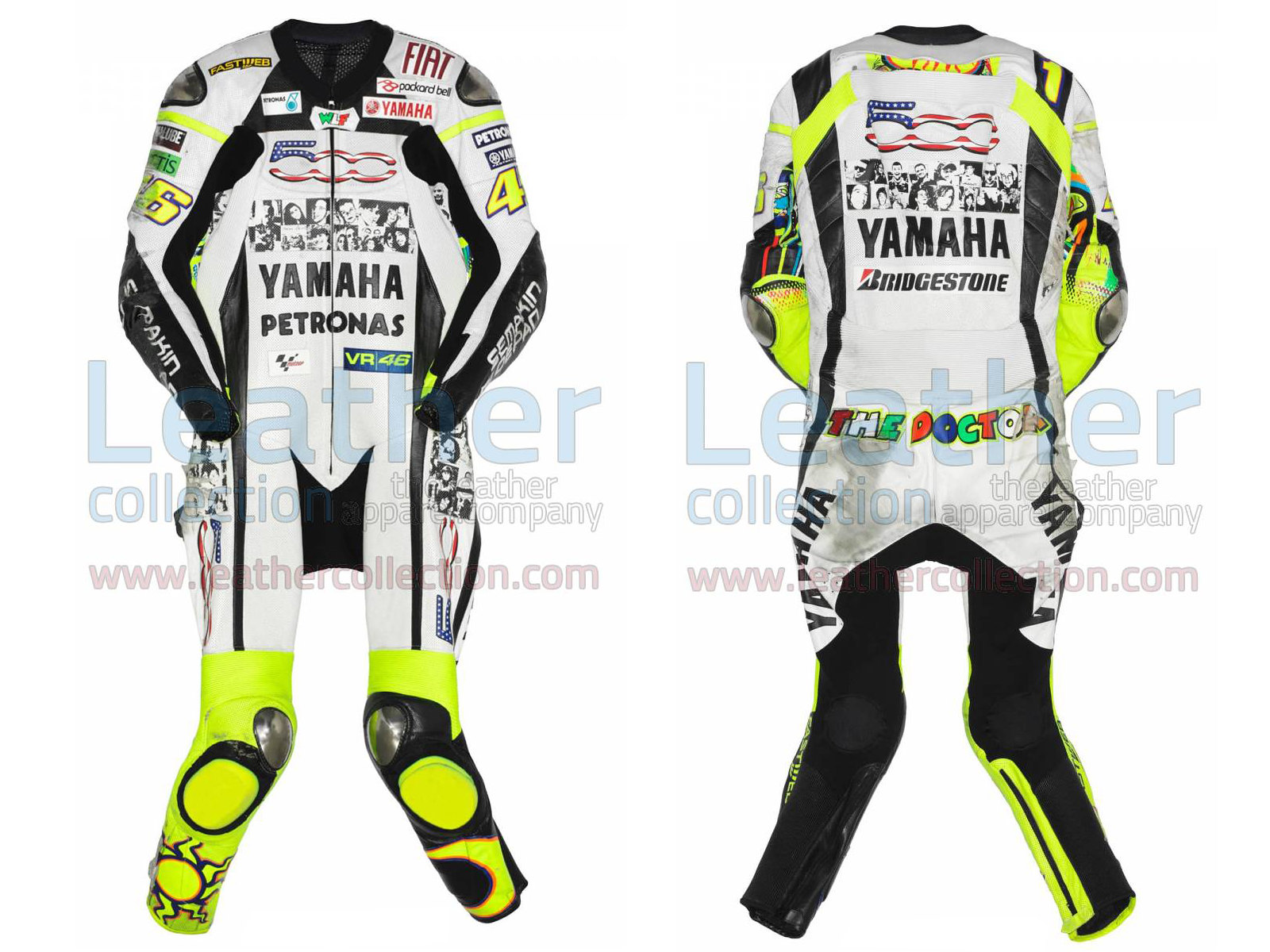The image showcases a front and back view of a leather motorcycle racing suit, predominantly white with black markings and neon yellow leg sections featuring black detailing. It prominently displays the names and logos of sponsors: "Yamaha" and "Petronas" on the front, and "Yamaha" and "Bridgestone" on the back, along with "The Doctor" written in multi-colored block capital letters across the waist or buttocks. The suit, designed with built-in knee pads and metal knee guards, also includes other sponsor logos such as Fiat and a number detailing, showing a 4 and a 6 on different sleeves. Additionally, the image features a watermark that reads "Leather Collection" and "The Leather Apparel Company," accompanied by a website URL: www.leathercollection.com.